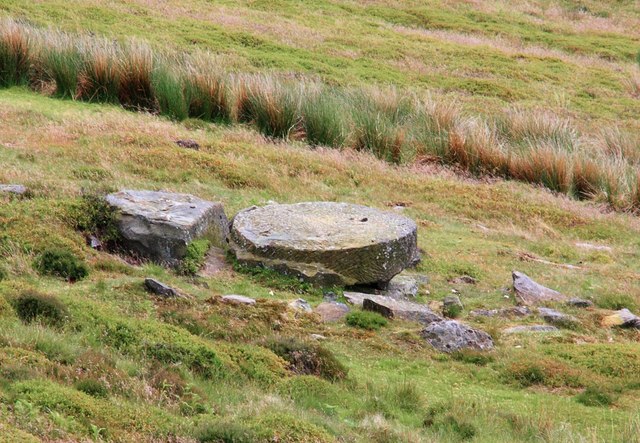The image captures a grassy hillside with a gentle slope, suggesting some elevation. The landscape features varying grass heights, with a row of taller, two-foot-tall grasses partly browned at the tops, suggesting late summer or early fall. The foreground is dominated by an intriguing, large circular stone, resembling a millstone or a wheel with visible carving marks, indicative of its handcrafted, potentially historical origins. Scattered around this central stone are smaller gray rock fragments, hinting at the remnants of a past settlement or structure. The scene, set in a natural, outdoor environment, depicts a mix of green, brown, tan, gray, black, and yellow hues under daylight, contributing to a serene and timeless atmosphere.